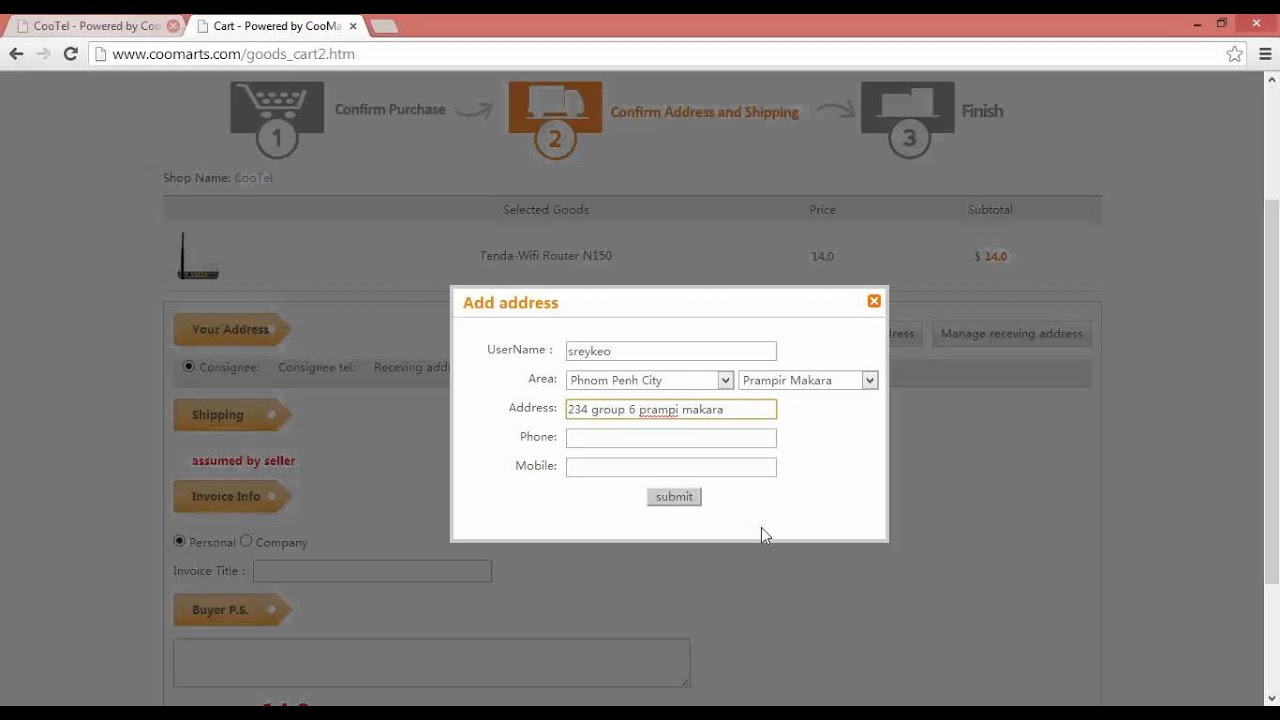This is a detailed screenshot of a webpage from www.qmarts.com, specifically at the URL "goods_cart2.htm," indicating the user is in the second step of a purchasing process. The screenshot features a central pop-up text entry box for adding an address. The page has a partially darkened background, suggesting a focus on the pop-up window. 

The purchasing process appears to have three steps, of which the user is currently on the second step, highlighted in orange and labeled "Confirm Address and Shipping." The previous step, likely confirming the purchase, is completed, and the final step, labeled "Finish," is yet to be completed.

Within the pop-up, the user is prompted to enter their address information. The displayed fields include:
- Username: srayko
- Area: Phnom Penh City
- District: Prampeer Makara
- Address: 234 Group 6, Prampeer Makara

Additional fields for "Phone" and "Mobile" numbers are present below the address information. At the bottom of the pop-up, there is a gray "Submit" button for confirming the entered details. This screenshot captures a step in the user’s process of providing their shipping information on the ecommerce website.